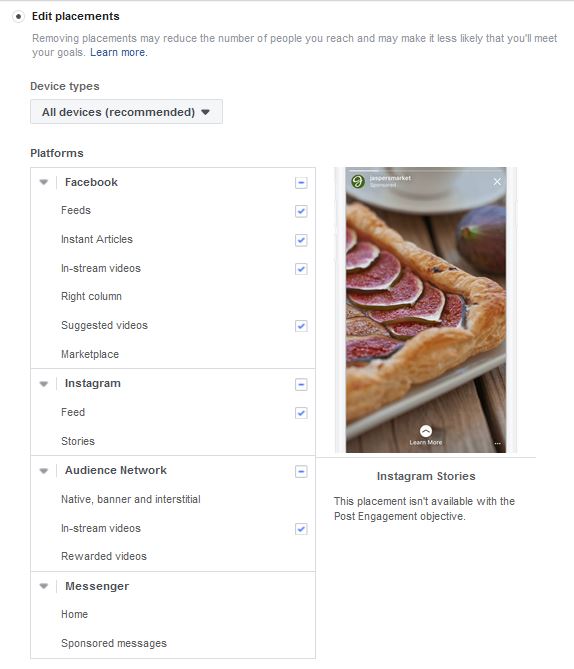This screenshot captures the backend interface of a website, specifically focusing on advertisement placements settings. At the top, there's a radio button labeled "Edit Placements." Beneath this, a warning message states, "Removing placements may reduce the number of people you reach and may make it less likely that you'll meet your goals," accompanied by a blue "Learn More" link for additional information.

Further down, there's a section titled "Device Types," featuring a dropdown menu with the option "All Devices (Recommended)" selected. 

Below this, in a category named "Platforms," there's a detailed list of platform-specific placement options, organized into expandable sections:

- **Facebook**: Includes feeds, instant articles, in-stream videos, right column, suggested videos, and marketplace.
- **Instagram**: Features placements for feeds and stories.
- **Audience Network**: Lists native, banner, and interstitial ads, along with in-stream videos and rewarded videos.
- **Messenger**: Offers placements in the home section and for sponsored messages.

To the right, there's an image preview of an Instagram post displaying a visually appealing type of pizza.